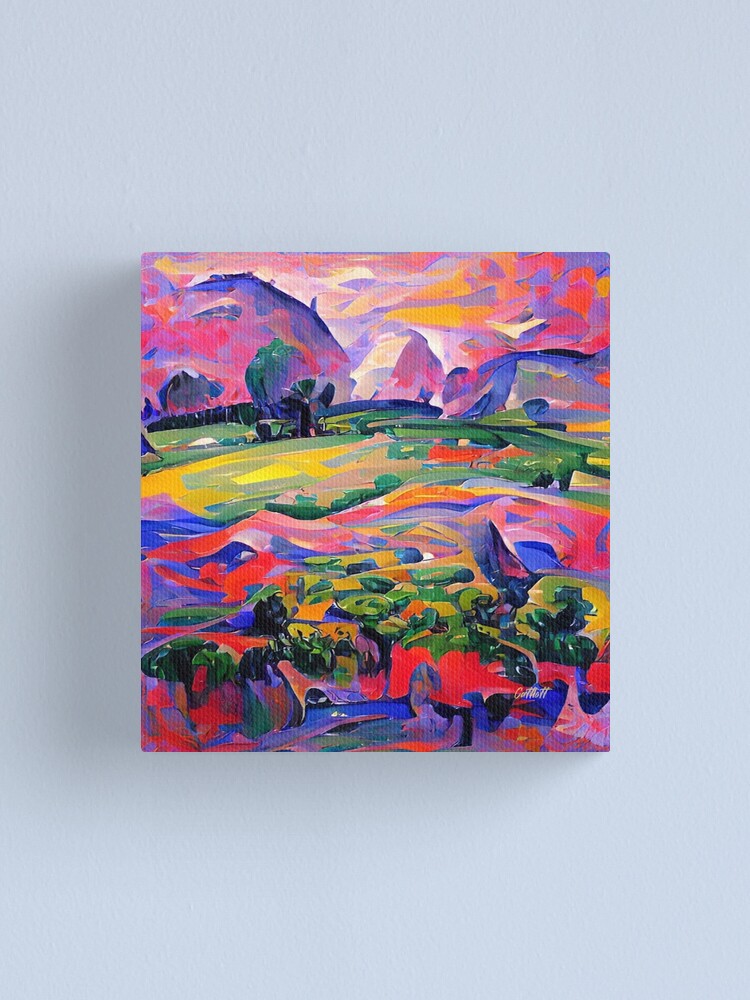This image features a vibrant and abstract watercolor painting hanging on a bluish-gray wall, unframed and presented on its canvas. The scene depicted is a colorful outdoor landscape, possibly a farm with mountains in the background. The foreground showcases an array of colors and brushstrokes that suggest bushes, trees, and potentially a house. The sky is painted with bright hues of pinks and purples, transitioning into blues, greens, yellows, and reds that blend together, creating a mosaic of colors across the entire canvas. The painting's abstract nature leaves the exact details open to interpretation, emphasizing the artist's use of vivid watercolors to create a dynamic, visually striking image.